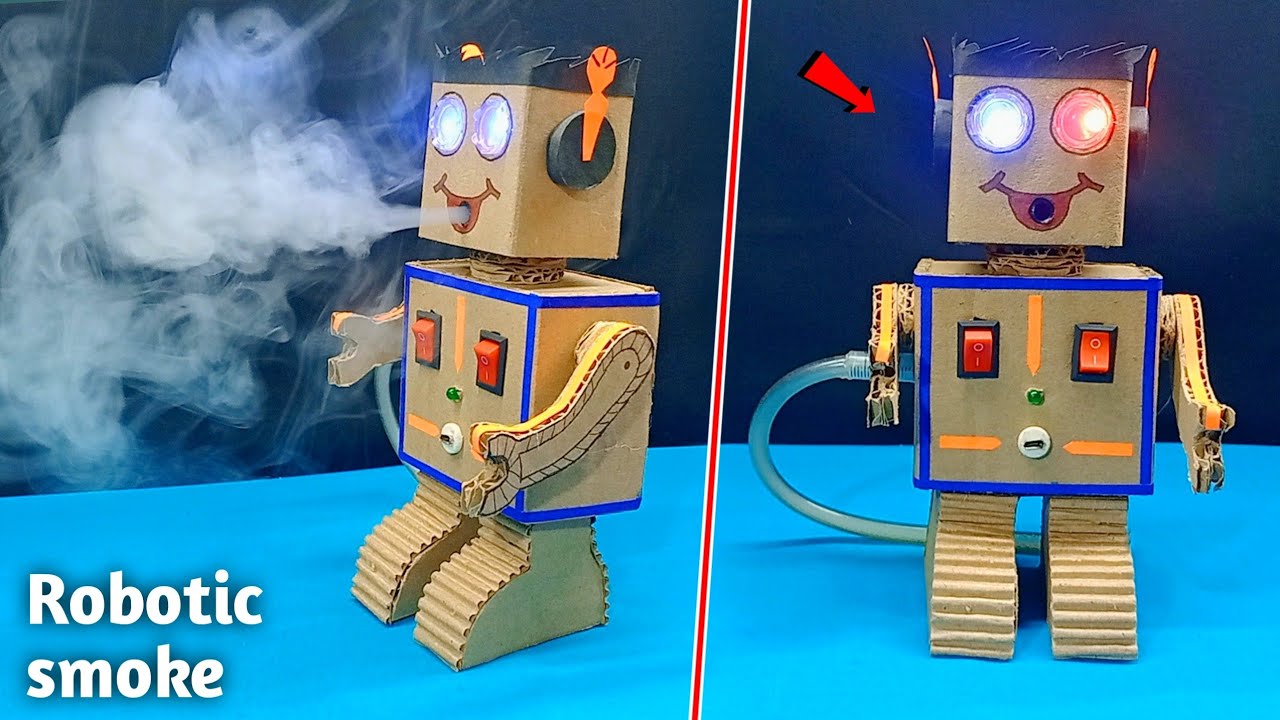The image depicts two side-by-side photographs of a rudimentary robot, seemingly made from cardboard and tape, with the left photo showing it from an angled perspective and the right photo from a head-on view. Both photos are adorned with the caption "Robotic Smoke" in the bottom left corner, featuring a red arrow pointing from the left image to the right image. In the left-hand photograph, the robot is facing to the left, expelling a billowing cloud of smoke from its mouth, which is a hole on its face. The robot has distinctive features: glowing red and blue eyes, black spiky hair, and a body fitted with two red and silver toggle switches and additional buttons. The right-hand photo provides a frontal view of the robot, where the smoke is not visible. A hose or tube attached to the back of the robot, likely the source of the smoke, is clearly visible. The chest also reveals wrench-like arms and the detailing of the cardboard construction, including the corrugated texture on its legs, suggestive of added traction.